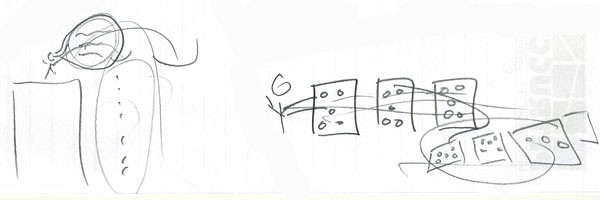The image is a detailed hand-drawn pencil sketch on a white piece of paper, which features a faint but discernible watermark with an upside-down "R-U-C-O" possibly reading "Rucco." The drawing predominantly occupies the upper half of the paper, centering around a tall, rectangular skyscraper.

Atop the skyscraper stands a stick figure with a large speech bubble, suggesting they are shouting. The speech bubble is filled with unintelligible scribbles, and notably, the words appear to be cascading down the building in an exaggerated manner, emphasizing the figure's outburst.

To the right of the skyscraper, another stick figure is seen supporting or interacting with an array of dominoes. This figure appears to be holding onto a single domino while the others lean nearby. The top three dominoes are clearly marked with the number five. The stick figure's hands are depicted as scribbles atop the dominoes. Below this row, a second series of dominoes is arranged, illustrating two with the number five and one with the number three, contrasting with the uniformity of the previous set.

The scene possibly portrays a narrative where the second stick figure's attempt to achieve a perfect sequence of five-marked dominoes has faltered, highlighted by the appearance of a three. This perceived failure leads the figure to the skyscraper's roof to express frustration or disappointment, dramatically illustrated by the descending speech bubble. The drawing captures a blend of simple figures and dynamic storytelling through its use of emotive scribbles and symbolic placement of objects.